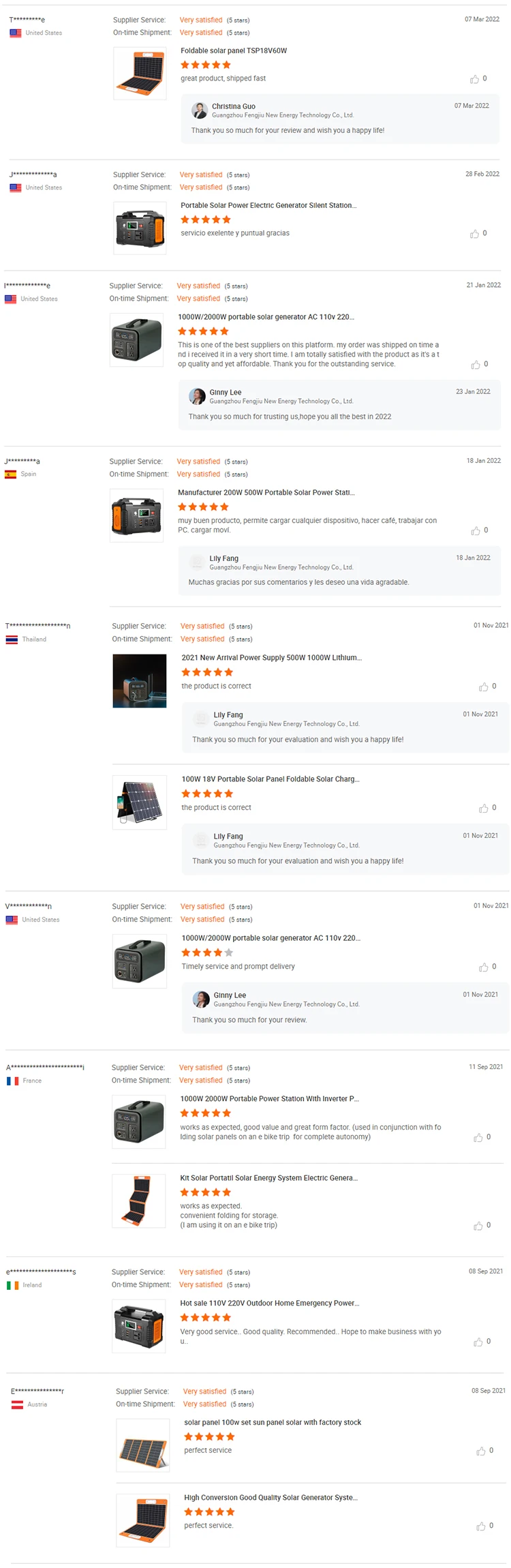This detailed caption gives a thorough description of a screenshot showing an international review section on an unspecified marketplace website. Each reviewer's name is partially obscured, displaying only the first and last letters. The reviews originate from various countries, including the United States, Spain, Thailand, France, Ireland, and Austria. The feedback pertains to a variety of products, with some items recurring occasionally amid the diverse selection. One common factor across the reviews is the high satisfaction ratings for supplier service and shipping time, both consistently receiving five-star ratings.

The first review highlights a foldable solar panel, specifying the product or model number, accompanied by a five-star rating and the comment, "Great product, shipped fast." In response, the supplier named "Goo" offers a gratitude-filled acknowledgment, saying, "Thank you so much." This pattern of detailed reviews and supplier responses continues for different items in the section, reflecting a robust and globally-representative feedback system.